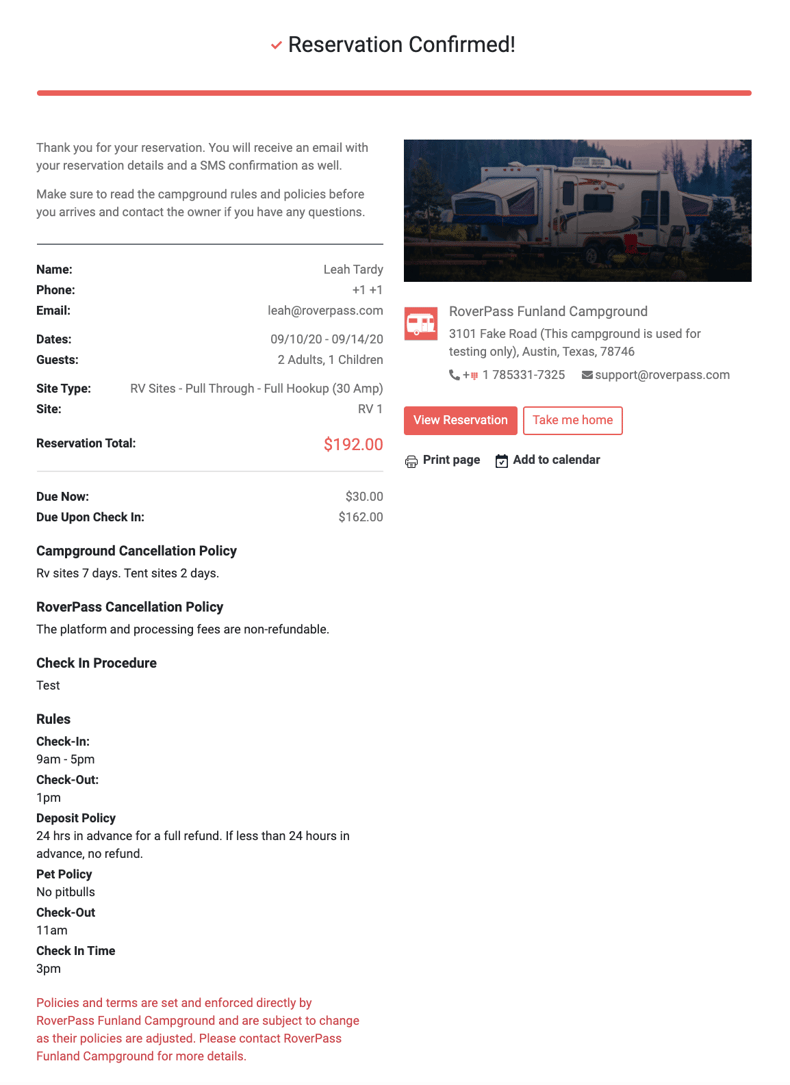The image depicts a reservation confirmation notice for a campground stay. At the top, there's a bold red checkmark next to the text "Reservation Confirmed." Below this, a horizontal red line separates the header from the main content. The notice features an image of a camper or RV, symbolizing the upcoming adventure.

The text reads: "Thank you for your reservation. You will receive an email with your reservation details and an SMS confirmation as well. Make sure to read the campground rules and policies before you arrive, and contact the owner if you have any questions."

Key reservation details provided include:
- **Name**
- **Phone**
- **Email**
- **Dates**
- **Guests**
- **Type**
- **Site**
- **Reservation Total: $192**

Additional information is given about various policies, including:
- Campground Cancellation Policy
- Check-In Procedure
- Campground Rules
- Check-In and Check-Out times
- Deposit Policy
- Pet Policy
- Check-In Time